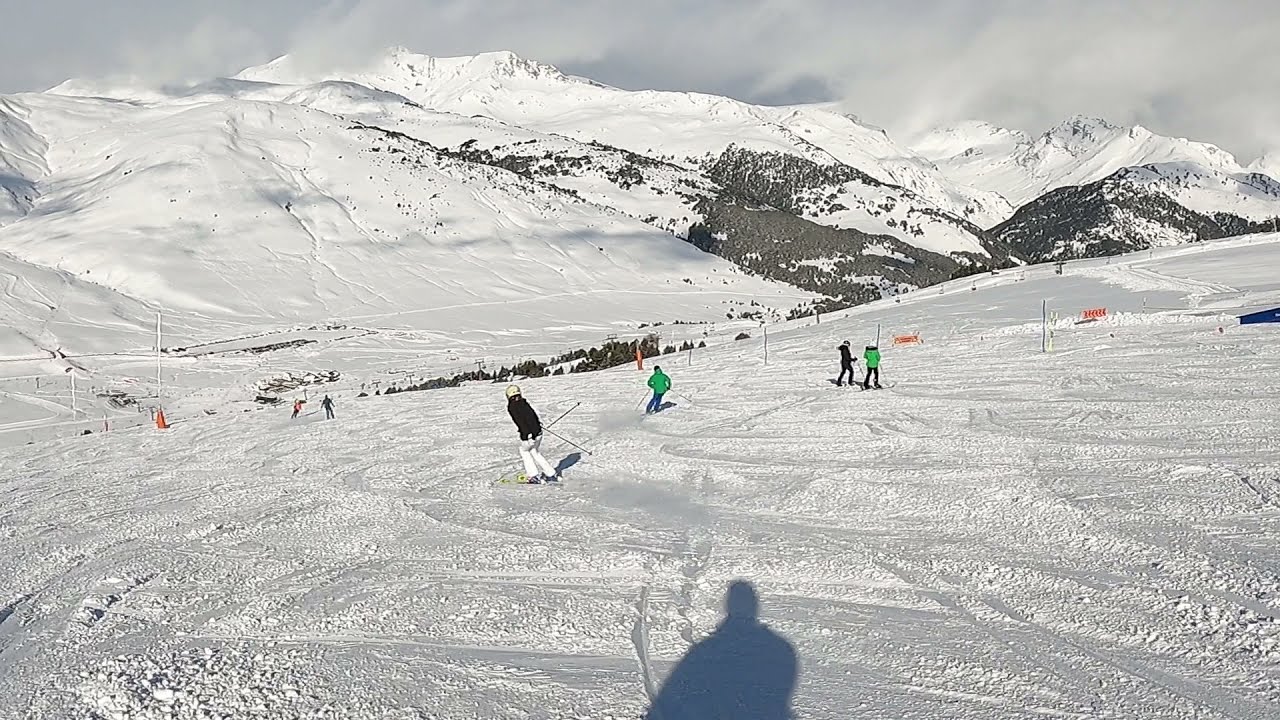This horizontally aligned rectangular image captures a wintry ski slope scene during the daytime. At the very top, the sky is gray, blending with several white clouds. The background reveals snow-covered mountain sides and peaks, with patches of brown terrain visible through the snow. In the foreground, the slope inclines slightly downward, featuring numerous skiers. At least six skiers are present, with two individuals standing still just off to the right—one dressed in green and the other in black. In the middle, a skier wearing blue pants and a green jacket is in motion, while to his left, another person sporting white pants, a black jacket, and a white helmet prepares to descend. Marks from previous skiers crisscross the snow, and faint shadows, including that of the person taking the picture, stretch out ahead. Midline on the right, some fencing is visible, while yellow cones on the mid-left side of the image mark the trail. The entire scene is enveloped in a crisp, snowy ambiance, enhancing the outdoor, mountainous setting.